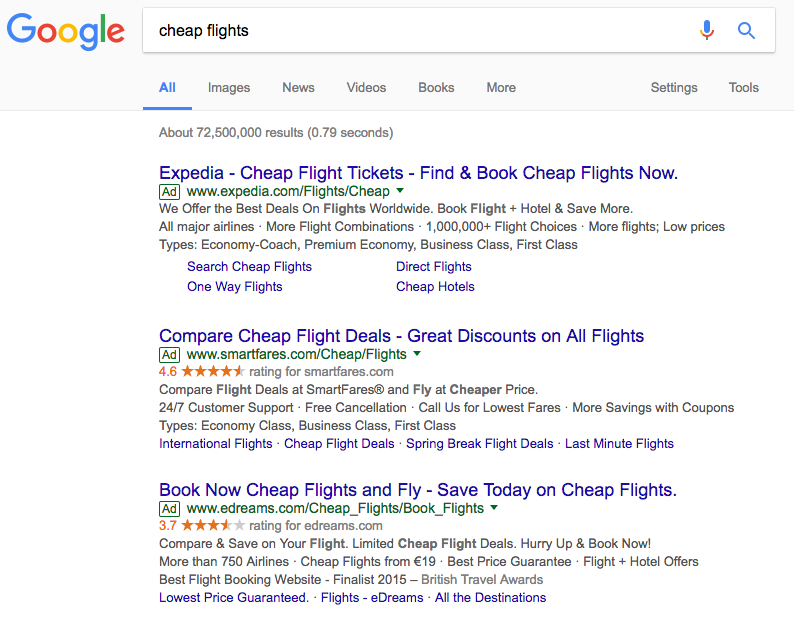The image depicts the Google search user interface, centering on a search query for "cheap flights." The search bar, within a gray box, displays the query next to a blue microphone icon with a hint of orange, and a blue magnifying glass icon. Above the search bar, the colorful Google logo is visible, with letters in blue, red, yellow, green, and red respectively. Below the search bar, a focused menu path highlighted in blue with an underline displays options: Images, News, Videos, Books, and More. To the right, additional options like Settings and Tools are visible.

The results section indicates approximately "72,500,000 results (0.79 seconds)." The first three entries are ads.

1. **Expedia Cheap Flight Tickets**:
   - URL: www.expedia.com/flights/cheap
   - Description: "Find and book cheap flights now. We offer the best deals on flights worldwide. Book flights plus hotel and save more. All major airlines, more flight combinations, 1 million+ flight choices."
   - Types: Economy Coach, Premium Economy, Business Class, First Class
   - Links: Search Cheap Flights, One-way Flights, Direct Flights, Cheap Hotels

2. **Smartfares Cheap Flight Deals**:
   - URL: www.smartfares.com/cheap/flights
   - Rating: 4.6 out of 5 stars (in orange text)
   - Description: "Compare flight deals at Smartfares. Fly at cheaper prices. 24/7 customer support, free cancellation. Call us for lowest fares, more savings with coupons."
   - Types: Economy Class, Business Class, First Class
   - Links: International Flights, Cheap Flight Deals, Spring Break Deals, Last-minute Flights

3. **eDreams Cheap Flights**:
   - URL: www.edreams.com/cheap_flights/book_flights
   - Rating: 3.7 out of 5 stars (in orange text)
   - Description: "Fly and save today on cheap flights. Compare and save on your flight with limited cheap flight deals. Hurry up and book now. More than 750 airlines, cheap flights from 19€, best price guaranteed, flights + hotel offers. Best flight booking website finalist in 2015 for the British Travel Awards."
   - Links: Lowest Price Guaranteed, Flights, eDreams, All Destinations

Each ad prominently features compelling offers, star ratings for credibility, and various flight types and categories, with clickable links for more specific searches.